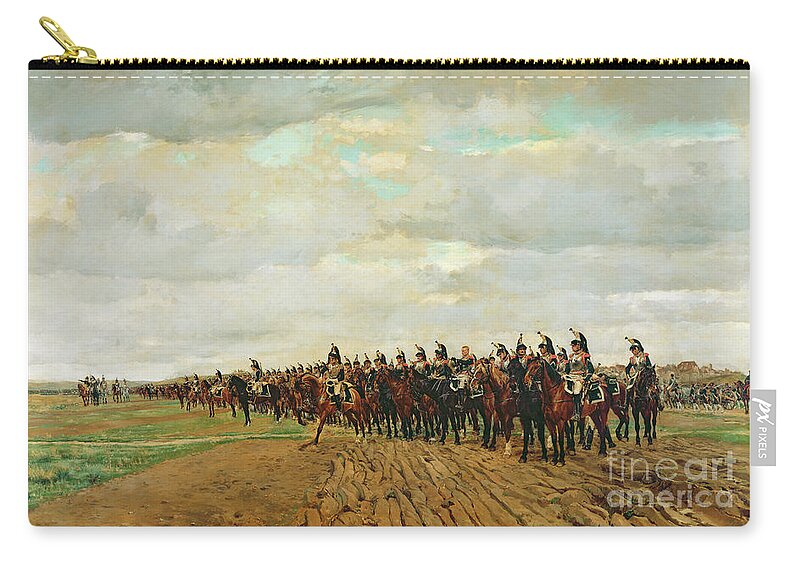The image depicts a small coin pouch featuring an intricately painted outdoor scene that portrays soldiers from the Napoleon era. The soldiers, clad in uniforms, are on horseback, with the majority of the horses being brown and black. The soldiers are aligned, appearing ready for battle, and some hold rifles. The scene extends from the right side of the pouch to the left, where they are waiting for their general in the far distance. The background reveals a field with brown grass and dirt, interspersed with green patches. On the right side, there are brown houses and a hill. The sky above the soldiers is filled with puffy clouds in shades of white, gray, and blue, with a hint of tan. The pouch has a black zipper at the top, complemented by gold stitching and a gold pull tab. The bottom right corner of the pouch reads "Fine Art America" in gray text. The detailed image is titled "The Coursers Before Their Charge."